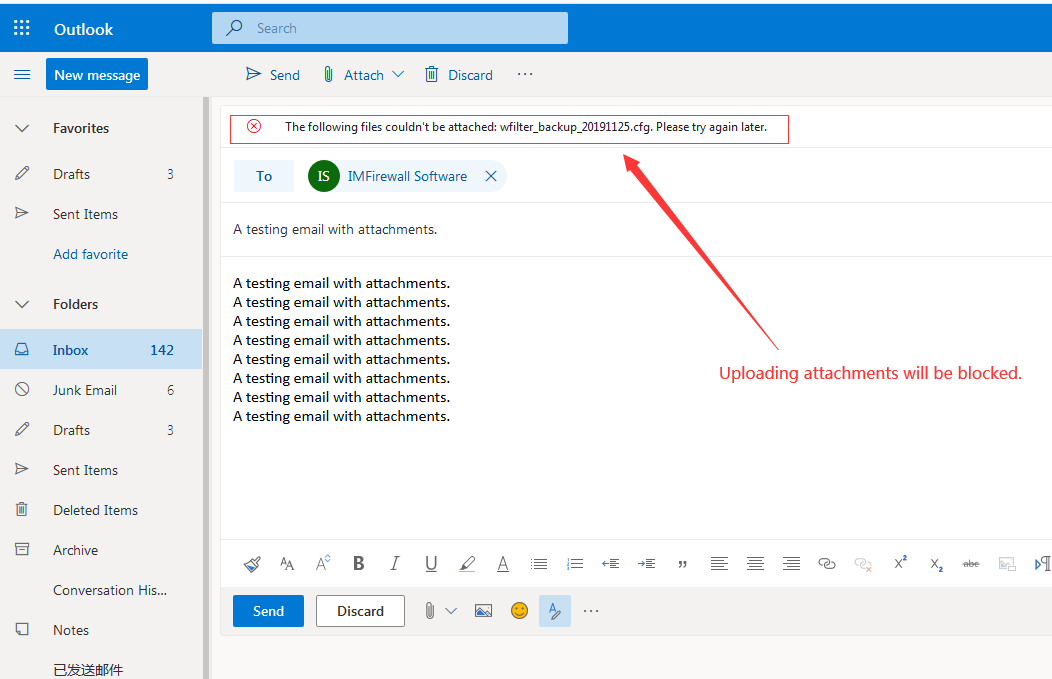In this image, an Outlook email composition window is open. The email is addressed to "IM Firewall Software" with the subject line "Testing email with attachments." The body of the email repetitively contains the phrase "a testing email with attachments," written eight times. A notification bar at the top, highlighted in red with a red 'X' mark, displays an error message stating, "The following files couldn't be attached," followed by "wfilter_backup_20191125.cdf. Please try again later." A prominent red arrow points to another warning in red text, "Uploading attachments will be blocked." The Outlook interface features a blue title bar and buttons labeled "New Message" and "Send" in blue, contrasting with the light gray background and black text of the email contents. The red error notifications and red arrow stand out sharply against this monochromatic backdrop. This image appears to be either a genuine error or a staged spoof highlighting a failed attachment upload attempt in Outlook.